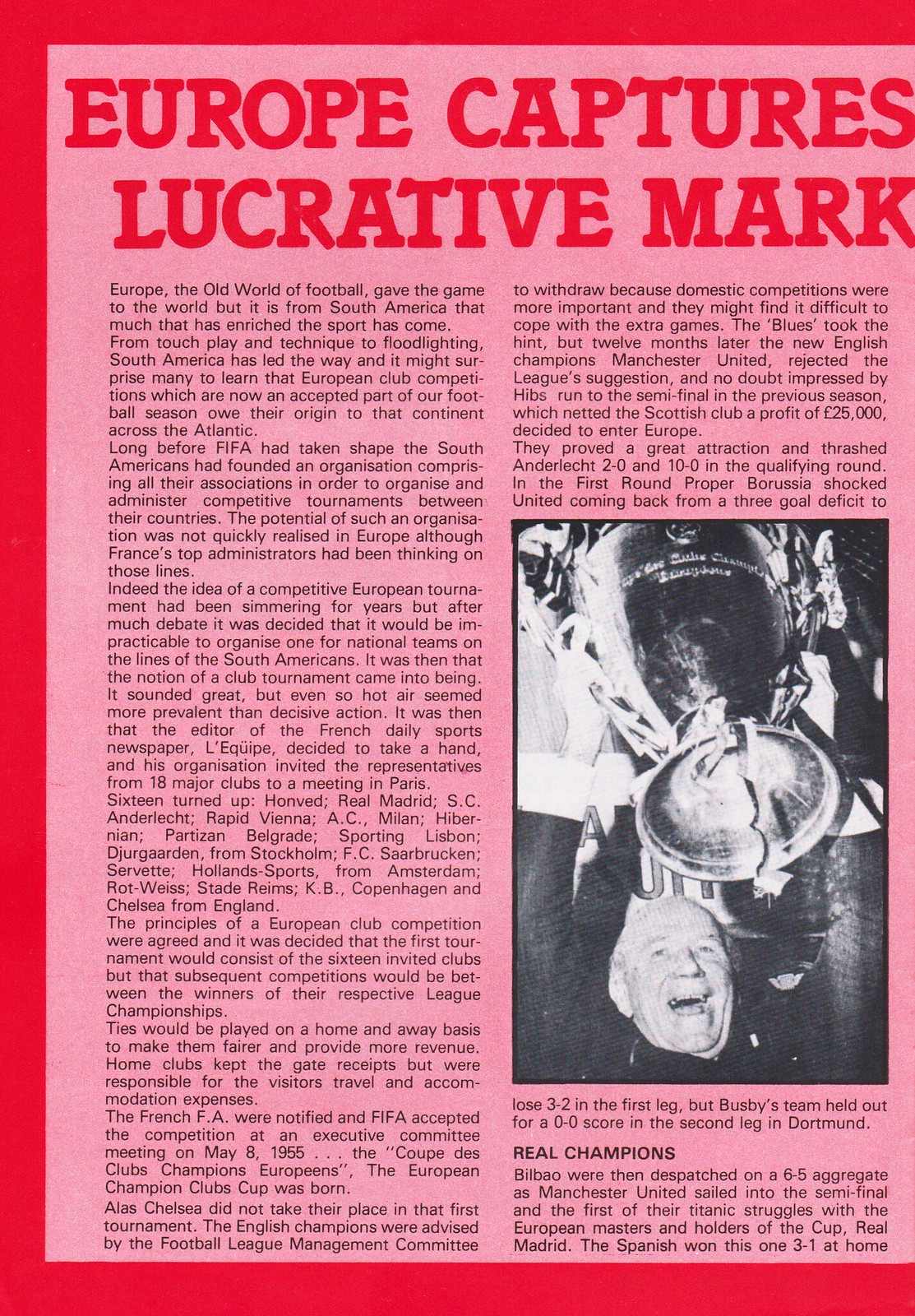The image depicts a vibrant magazine article with a light pink background and a striking thick red border. Bold red text at the top reads, "Europe captures lucrative mark." The article consists of two long columns of black and white print discussing the profound influence of South America on the sport of football, juxtaposed with its European origins. On the right side, an inset black and white photograph features an older gentleman, possibly a coach, jubilantly raising a large trophy cup, commemorating a significant victory. The image captures a moment of triumph and celebration within the sport, emphasizing the championship's importance.